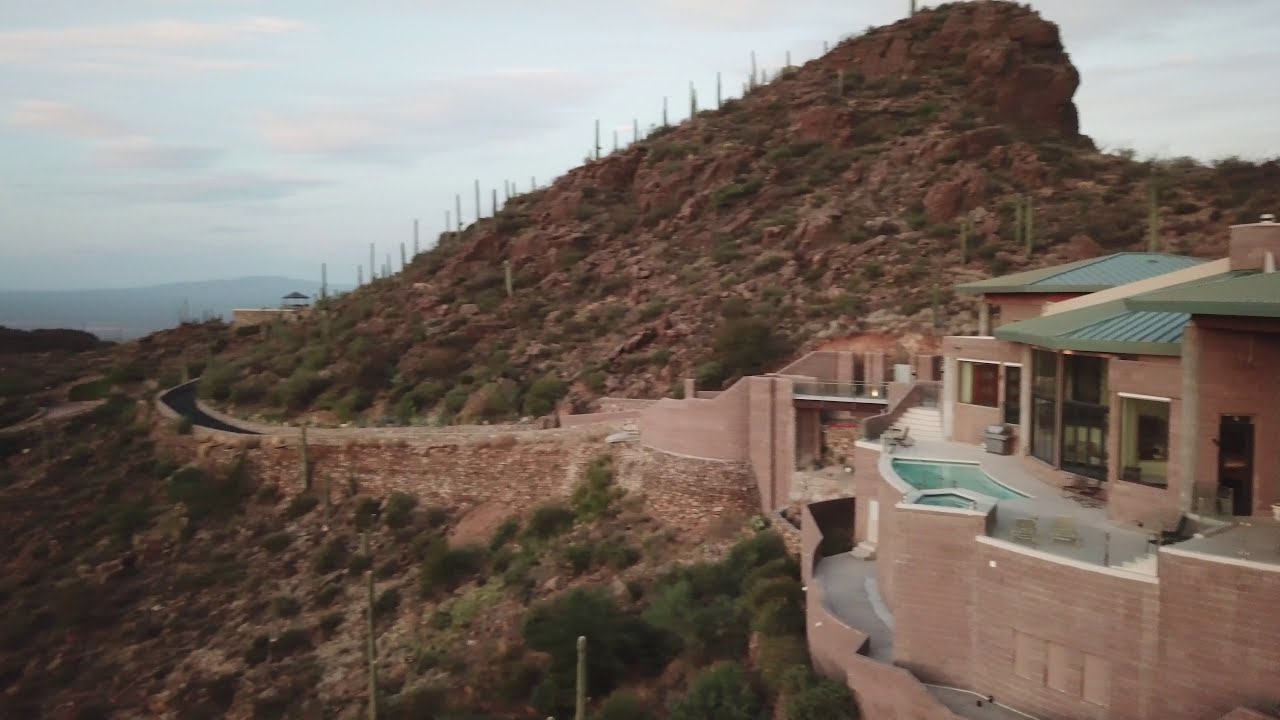This is a horizontal, rectangular photograph showcasing a luxurious landscape near a large body of water. The image features a striking, expensive-looking house on the right side, elevated from the ground with a large retaining wall in the back. The house has a beautifully landscaped backyard with an infinity pool, extending elegantly to the edge of the property. Adjacent to this house, there's another equally upscale residence, both sporting distinct green, brick roofs.

A dark, nicely paved private road, constructed from bricks, curves along the mountainside and extends from the left to the right side of the photo, leading toward the water. Lining this road, tall and slender cactuses add to the charm of the desert-like atmosphere, which suggests an Arizona setting. However, the area appears to receive a reasonable amount of rain, as evidenced by the green plants and bushes scattered throughout the landscape.

In the upper right corner, a uniquely shaped hill, sparsely populated with rocks, bushes, and few trees, rises above the scene, contributing to the dramatic terrain. The same type of land slopes downward on the opposite side of the road, emphasizing the rugged beauty of the surrounding environment.